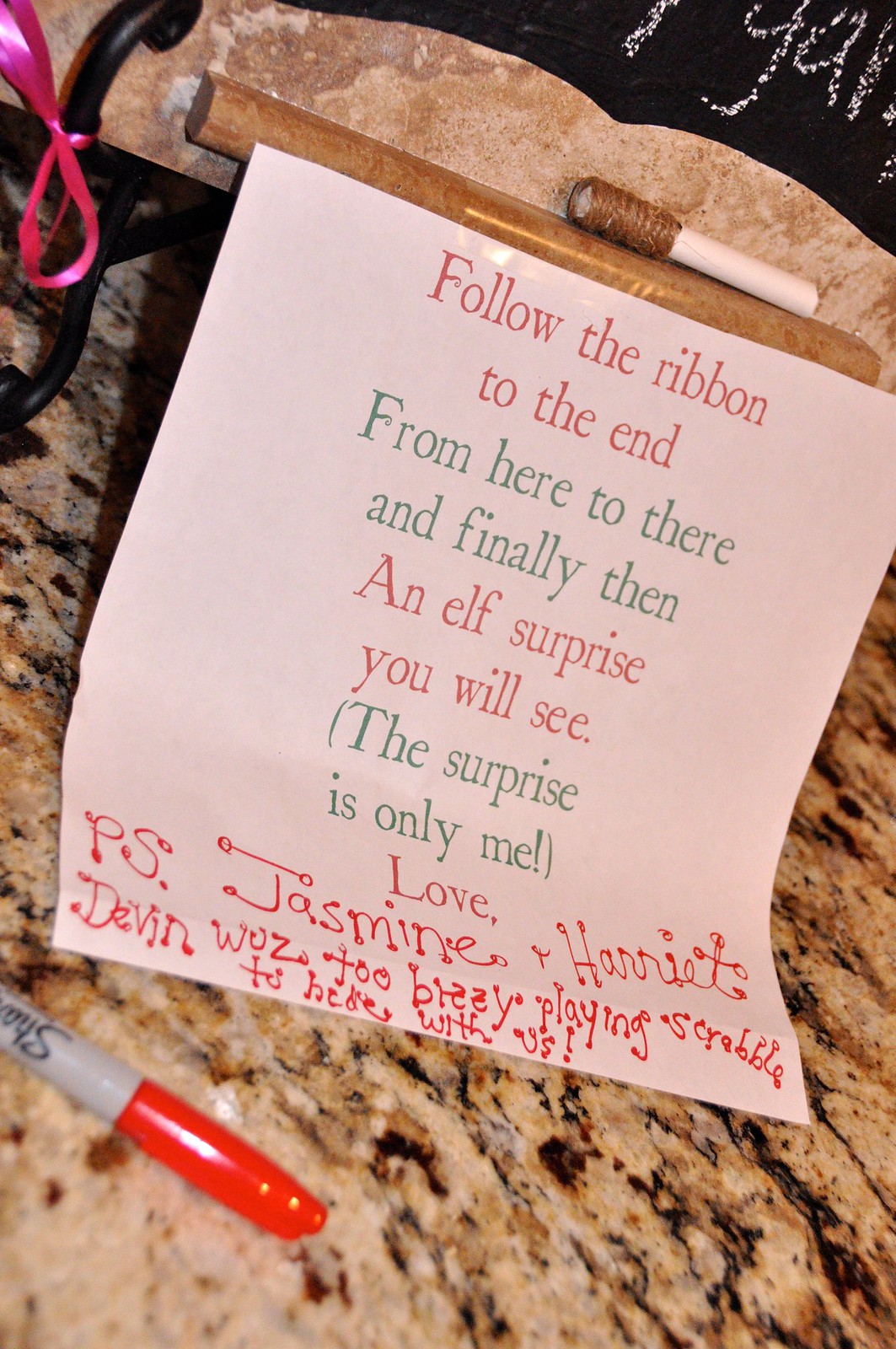The photograph, rectangular in shape, captures a note taped to the backsplash of what appears to be a kitchen setting. The backsplash and countertop underneath exhibit a stylish marble/granite finish in shades of browns, golds, blacks, and cream. Tied to the top left corner where the note is affixed, a pink ribbon is visible. Below the note, lying on the countertop, is a red Sharpie pen, although one description mistakenly identified it as grey with a red lid. The note itself is composed on a white piece of printer paper, featuring printed text in red and green that reads: "Follow the ribbon to the end, from here to there and finally then an elf surprise you will see. The surprise is only me." Beneath, handwritten in red Sharpie, it states: "P.S. Jasmine and Harriet, Devon was too busy playing Scrabble to hide with us." The entire arrangement is set against the textured, elegant background of the marble countertop.